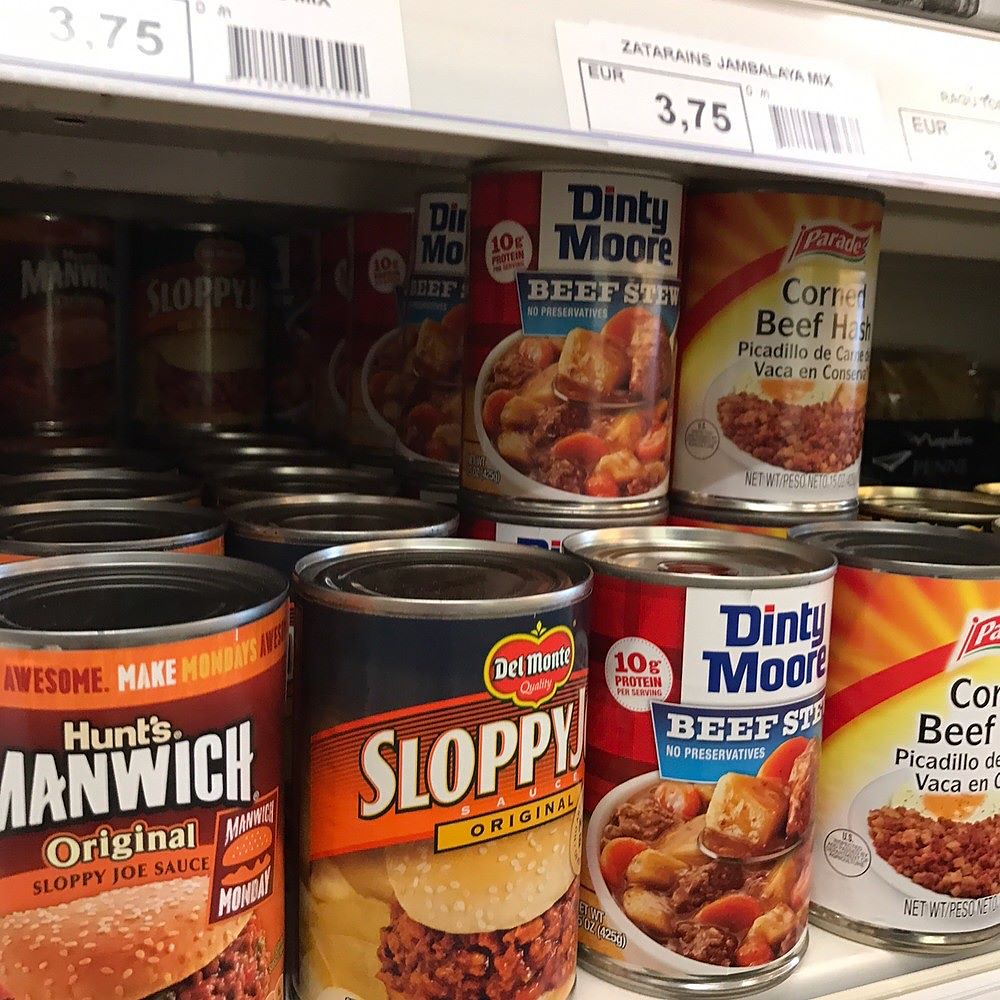This photograph showcases a grocery store shelf laden with various canned food items. At the top of the image, a white shelving unit is adorned with price stickers, visibly marked with black writing that indicates a price of $3.75 and features a barcode. On the lower portion of the shelf, a neatly organized array of canned goods is displayed. There are multiple cans of Hunt’s Manwich Original Sloppy Joe Sauce and Del Monte Sloppy Joe Original. Additionally, the shelf holds double-stacked cans of Dinty Moore Beef Stew and Parade Corned Beef Hash. Each item is meticulously arranged, offering a clear view of the brands and their respective labels.